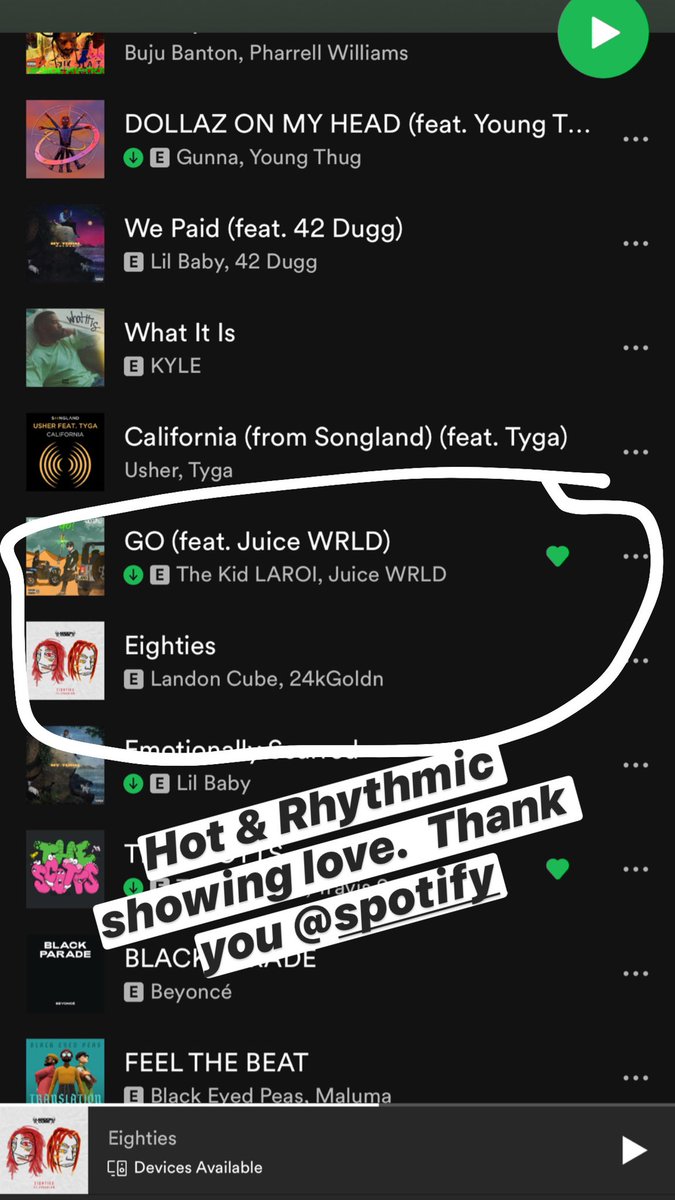The image displays a cell phone screen with a predominantly black background. A white, irregular oval has been hand-drawn around specific text, as if marked with a digital pen tool. Inside the circled area, you can read details about a music lineup: it mentions "Go (feat. Juice WRLD)" by The Kid LAROI, Juice WRLD, and "80s" by Landon Cube and 24kGoldn. Overlaid on the image are white rectangles with black text, which read "Hot and Rhythmic, Showing Love, Thank You," followed by "@Spotify" with "Spotify" in lowercase and underlined in black. At the bottom of the screen, text indicates "Devices Available" alongside an arrow pointing to the right.